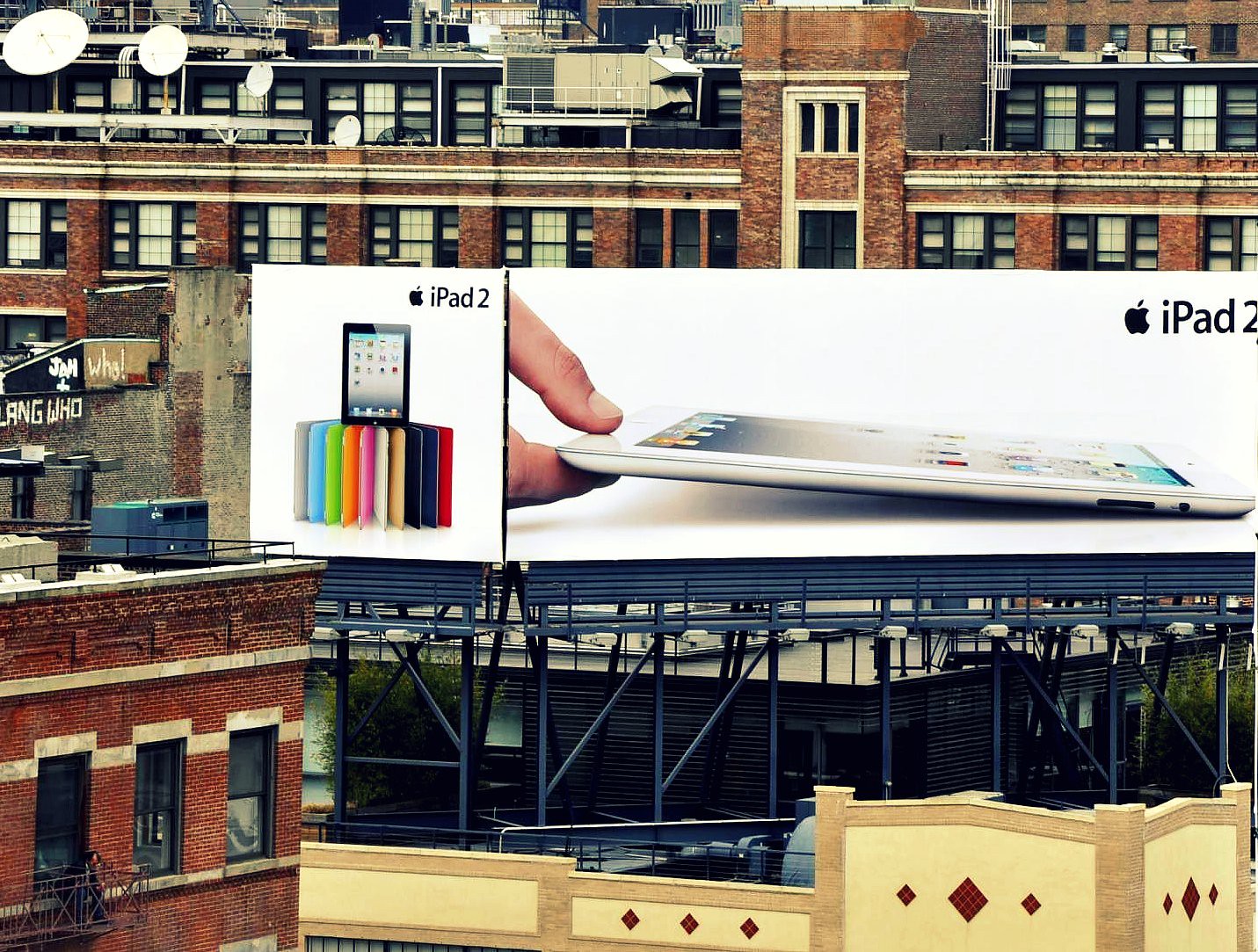The image captures a bustling downtown urban scene, characterized by predominantly brick buildings. The prominent structure in the background is a long, two-story office building adorned with a central tower. This building features light-colored cornices and window sills, and its roof is equipped with several communication dishes. In the foreground, another brick building is visible, sporting a metal fire escape that echoes the design of the rear office structure.

Closer to the viewer, a building with an angled roof is notable for its graffiti, which reads "JAH PLUS, Lang Hu, Hu!" in white spray paint. This graffiti-laden building contrasts against a nearby structure with a diamond-shaped facade in yellow and brown hues. Behind this facade, a tank is partially visible.

Prominently displayed are two billboards. The first, a double billboard, showcases an iPad 2 prominently placed over a series of fanned-out covers in various colors. Beside it, the second rectangular billboard features a close-up image of a hand, specifically a thumb and forefinger, placing the iPad 2 down on a white counter. Together, these elements create a vivid snapshot of urban commercial advertising amidst the architectural character of the downtown area.